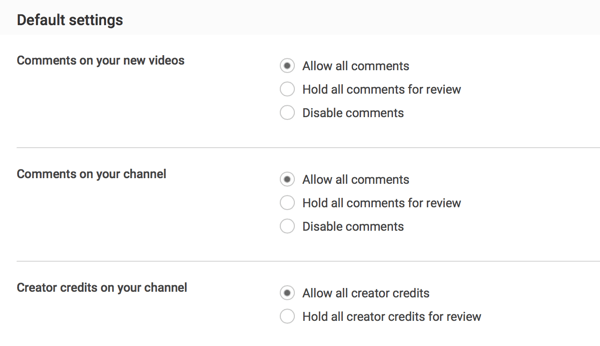This image is a detailed screenshot of a settings page on a YouTube channel, specifically focusing on comment and creator credit settings.

At the top left, the title "Default settings" is prominently displayed, followed by three subsections outlined underneath. These subsections are titled: "Comments on your new videos," "Comments on your channel," and "Creator credits on your channel." Each subsection is visually separated by horizontal lines, providing clear distinction between the categories.

To the right of the "Comments on your new videos" and "Comments on your channel" sections, there are three selectable options indicated by radio buttons. These options are: "Allow all comments," "Hold all comments for review," and "Disable comments." Currently, "Allow all comments" is selected, suggesting it is the default setting for these categories.

The "Creator credits on your channel" section at the bottom offers two options: "Allow all creator credits" and "Hold all creator credits for review." Unlike the comment sections, this setting does not provide an option to completely disable creator credits, reflecting an emphasis on ensuring proper attribution.

Overall, the page appears to be designed for users to manage how comments and creator credits are handled on their YouTube channel, emphasizing an element of control over interaction and attribution on their content.